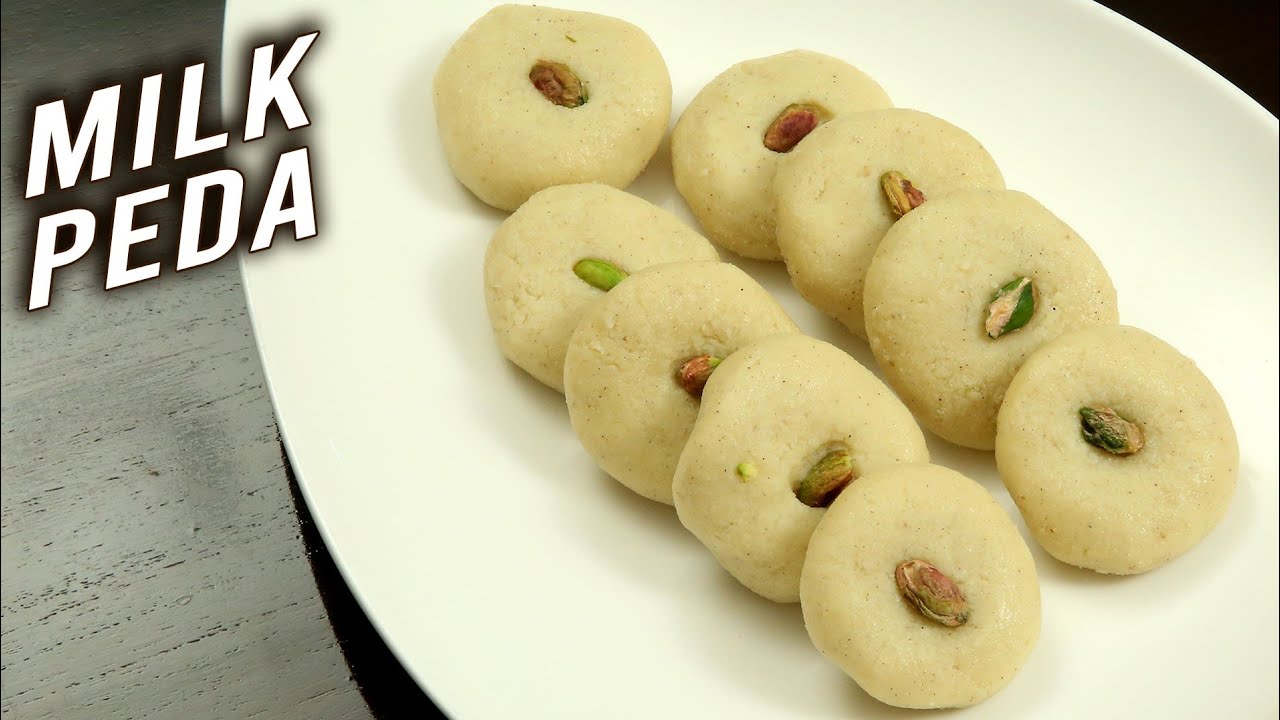The high-definition image showcases a delectable presentation on an off-white, oval-shaped platter. Positioned on a grayish wooden surface, the platter holds an array of nine cream-colored, circular cookies, neatly arranged in a pattern. Each cookie features a pistachio or similar nut in its center, giving them a rich, slightly greenish-brown appearance. The cookies are methodically placed in three rows, with some overlapping slightly. In the upper left corner, the image has text in bold, white font with a subtle drop shadow, reading "MILK PEDA," indicating this is an Indian sweet dish. The lighting source from the right accentuates the texture and details, making it a visually enticing photo likely intended for a social media or a food blog post.